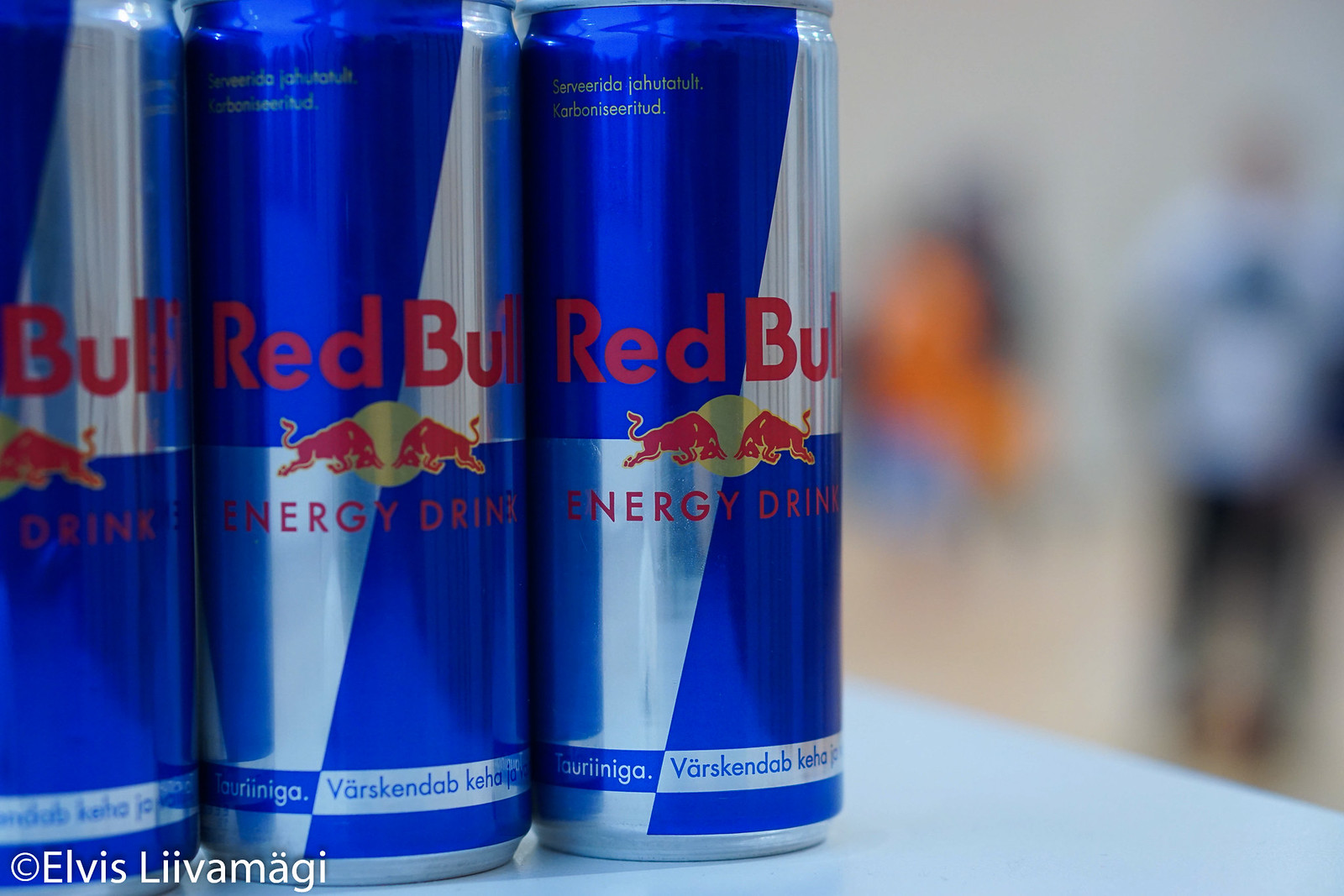In this close-up image, we see three Red Bull energy drink cans positioned on a light blue table. The cans, arranged from the middle towards the left side of the image, feature Red Bull’s iconic blue and silver diagonal split design. The text "Red Bull Energy Drink" along with the logo depicting two red bulls butting heads beneath a yellow sun is clearly visible. The can on the far left is partially cut off, revealing only the word "Bull." At the bottom left corner of the image, the words "Elvis Live Emoji" are inscribed, and below them, a copyright notice reads "© Elvis Liivamägi." In the blurry background, indistinct shapes of people can be seen, some appearing to wear red backpacks or other orange items.